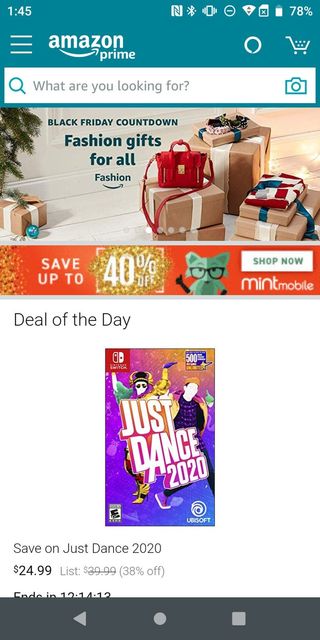The image features a clean, white background. At the top, there is a blue header displaying the text "145" alongside a battery icon indicating 78% charge. Next to it are three white lines and an Amazon Prime logo, followed by a small white circle and a white shopping cart icon. Below this header, there is a white search box.

Beneath the search box, there is a promotional banner with the headline "Black Friday Countdown: Fashion Gifts for All," showcasing several small packages and a woman's purse. To the left of this arrangement is a small Christmas tree, adding a festive touch.

Further down, there is a prominent red box that highlights a deal: "Save Up to 40% on Mint Mobile." This section also includes a "Shop Now" button for immediate action.

Continuing downward, the white background presents an advertisement for the game "Just Dance 2020." The game cover features a vibrant color palette of purple, orange, yellow, and green, with people dancing on the front. The text accompanying the image reads, "Save on Just Dance 2020, $24.99." A note indicates that this deal ends on December 14, 2013.

Finally, at the bottom of the image is a gray box containing a triangle, circle, and a square icon, possibly related to interactive elements or additional navigation options.